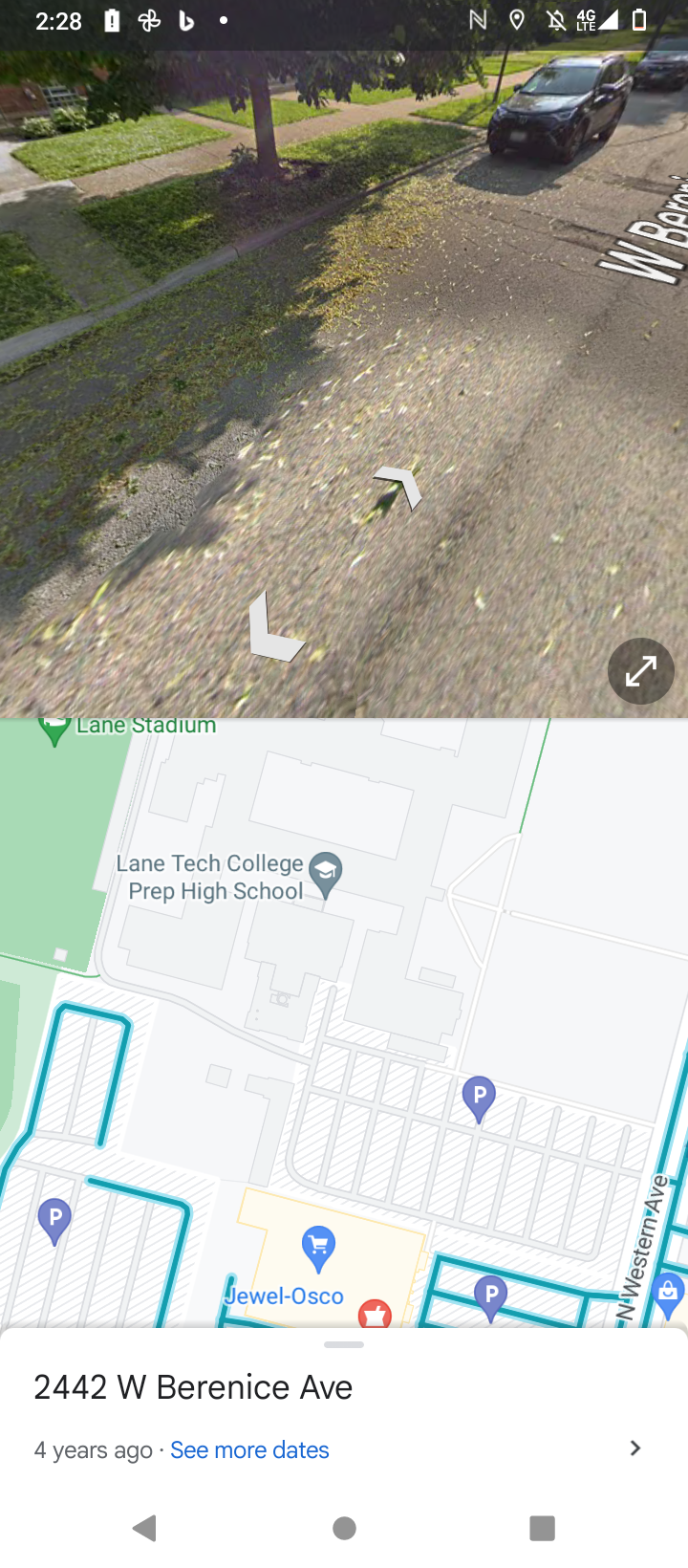The photograph shows a detailed street view captured by Google Street View, likely viewed on a smartphone with a low battery, as indicated by various notification icons at the top. The primary image depicts a dark gray road scattered with yellow and light green leaves. Prominent in the scene are the white directional arrows pointing left and right and the partially visible street name, which starts with "WBER." Further details reveal the full designation as 2442 West Bernice (or Baronice) Avenue. Parked along the street are a black car followed by a maroon one. The setting includes rectangular grass sections and circular mulch areas, each with large trees featuring dark green leaves and robust trunks. Sidewalks extending towards residential houses are also visible.

Directly beneath the street view is a bird's-eye map, highlighting the vicinity near Lane Tech College Prep High School, as well as nearby parks, various marked buildings in bright blue, a green-shaded stadium named Lane Stadium, and a shopping area indicated by a trolley icon. The map is part of what appears to be a Google Maps request made approximately four years ago, offering additional context to the location depicted in the street view above.